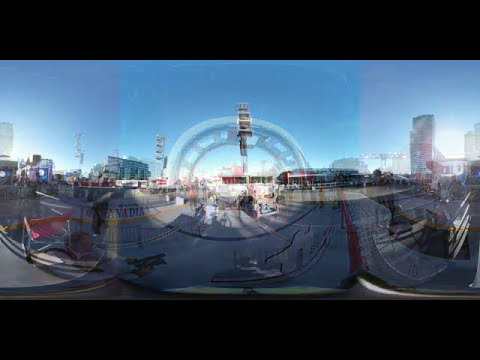The image, which appears to be taken through a glass window and is somewhat blurred, presents a complex urban scene. It's vertically oriented with black horizontal stripes at the top and bottom framing the image. In the background, various tall concrete buildings of different heights and shapes dominate the skyline. A large, somewhat blurry metal archway stands in the center, possibly a bridge or significant structure, giving the scene a focal point. Below the buildings, a paved road is visible, and the left side of the image shows what looks like a gray concrete walkway. There are reflections on the glass, indicating the photo was taken from inside a car or house, adding to the complexity of the scene.

On the right side, the image contains details such as a small bridge with a metal handrail and some people, including a man holding what could be a filming camera or a large object. There is also a red outdoor umbrella and a potential picnic table, suggesting an outdoor area. Additionally, there is a red bench with white wire-framed seating. To the left, a ship-like object suggests a harbor or waterfront area with shadows adding to the ambiguity. You can also see partial images of posters, with visible letters spelling "A-N-A-D-I-A," and a portable chair. There are numerous items superimposed and layered, making the image busy and filled with urban elements.